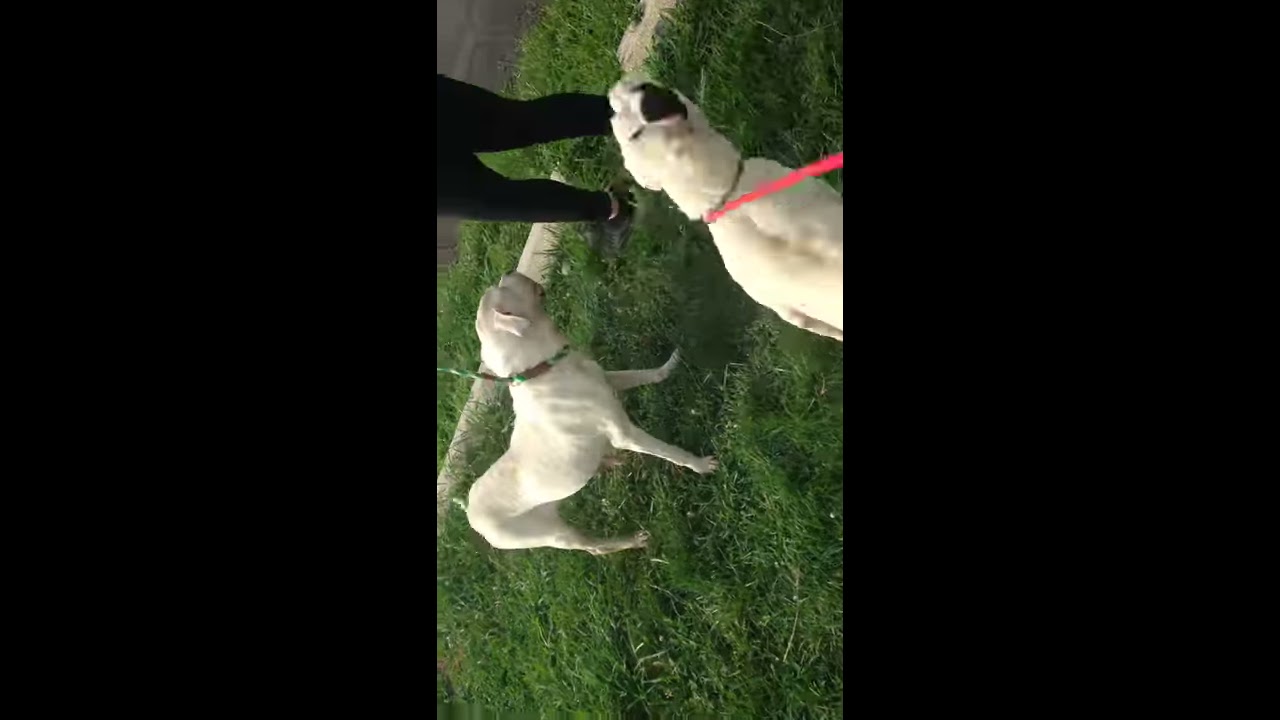This horizontally aligned, sideways-tilted image, framed by thick black borders, captures two medium-sized white dogs standing on a vibrant green lawn. The dog on the left, featuring a green and brown leash attached to a matching collar, appears to be focused on its handler. The dog on the right, distinguishable by a pink leash and a dark collar, has a striking black patch on its right ear while its left ear remains white. Both dogs are on leashes and near a person, whose only visible parts are the tight black leggings and black shoes, suggesting a female presence. The setting extends from this lush grass to an adjoining edge that transitions into asphalt, possibly a road or parking area, hinting at a varied terrain. The overall lighting indicates a dim, possibly overcast day, adding a subdued tone to the scene.